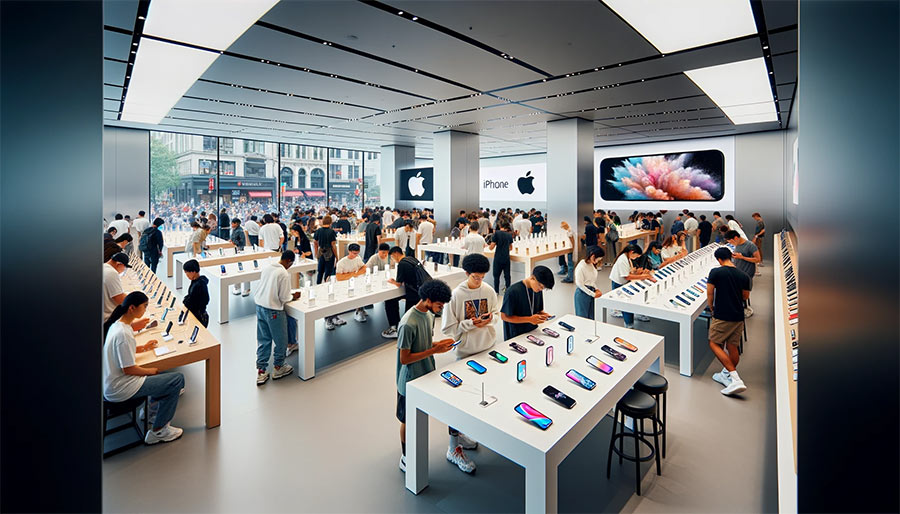This image captures the bustling interior of an Apple Store. Overhead, gray ceiling panels interspersed with black trim house modern, sleek lighting fixtures, casting a bright glow over the entire space. The walls are also painted a matching gray, adorned with the iconic Apple logos and symbols in pristine white and striking black.

In the top right corner, a large display showcases an Apple phone against the wall. Throughout the store, multiple tables are meticulously arranged, each serving its unique purpose. On the left side of the image, a long brown table features several people seated with various devices in front of them, fully immersed in their activities.

The center section of the store is dominated by white tables, each displaying an array of Apple devices. Customers are seen eagerly interacting with the gadgets; some are holding the devices, while others are intently observing them as they rest on the tables.

In the top left area, the glass storefront is visible, allowing natural light to blend seamlessly with the interior lighting. Below some of the tables, a series of black-colored stools are placed, with individuals seated on them, engaged in conversation or consumed by their devices. The store's floor is a light gray, seemingly composed of tile or stone, adding to the clean, modern aesthetic typical of Apple Stores.